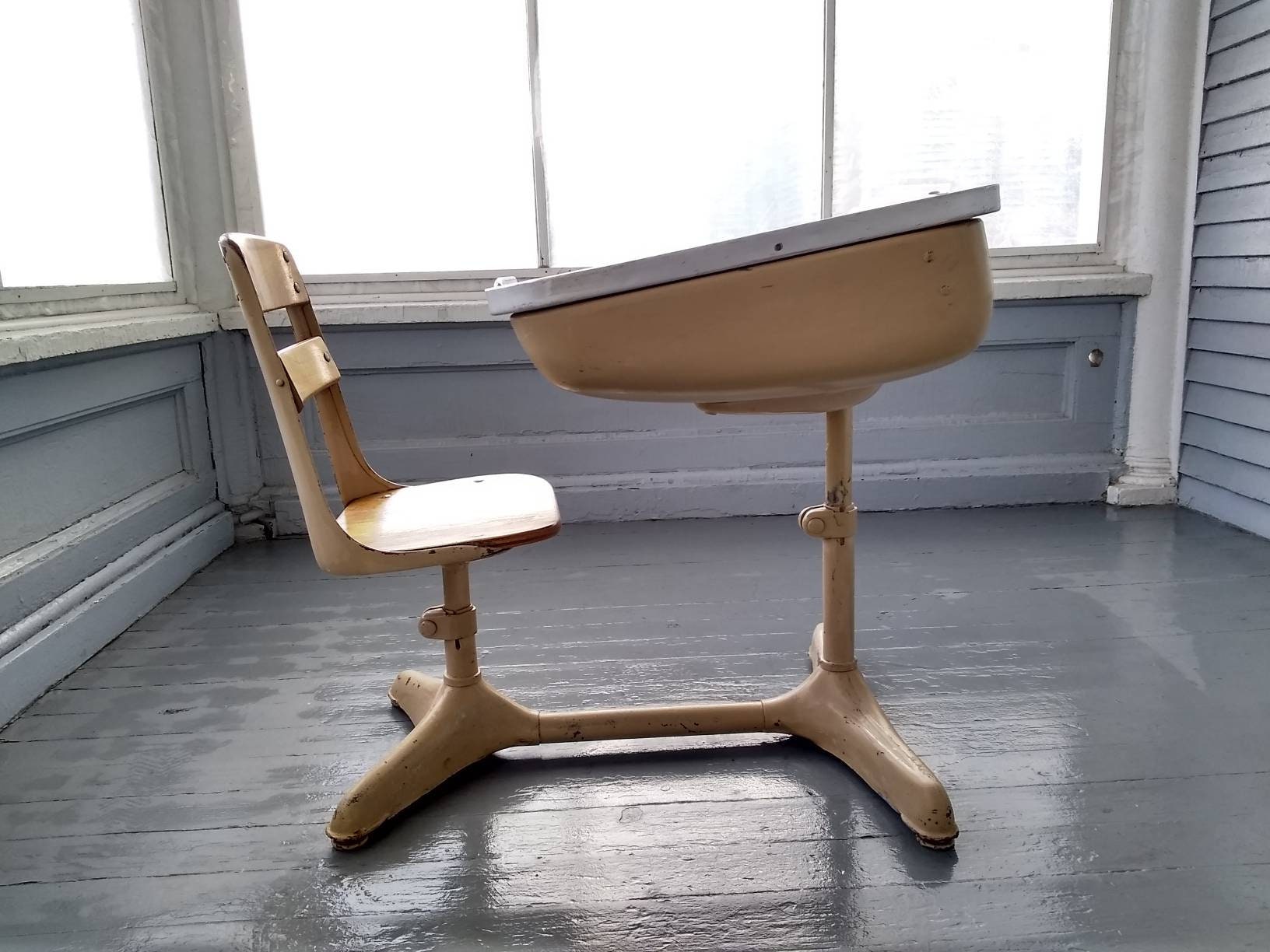The image depicts a vintage school desk, designed for a preschooler or kindergartener, situated in the corner of a room. This old-fashioned desk, combining a wooden seat and backrest with a beige metal frame, also features a slanted, white metal top that opens to reveal a storage compartment. Its positioning suggests it's directly in the middle from one perspective, flanked by windows on the left and behind it, casting natural light across the scene. The floor and walls of the room have a bluish-gray hue, with the walls adorned with wooden panels or slats, giving an antique feel to the overall setting. The room’s decor, including the painted gray floor, emphasizes the historical and nostalgic ambiance of the scene.